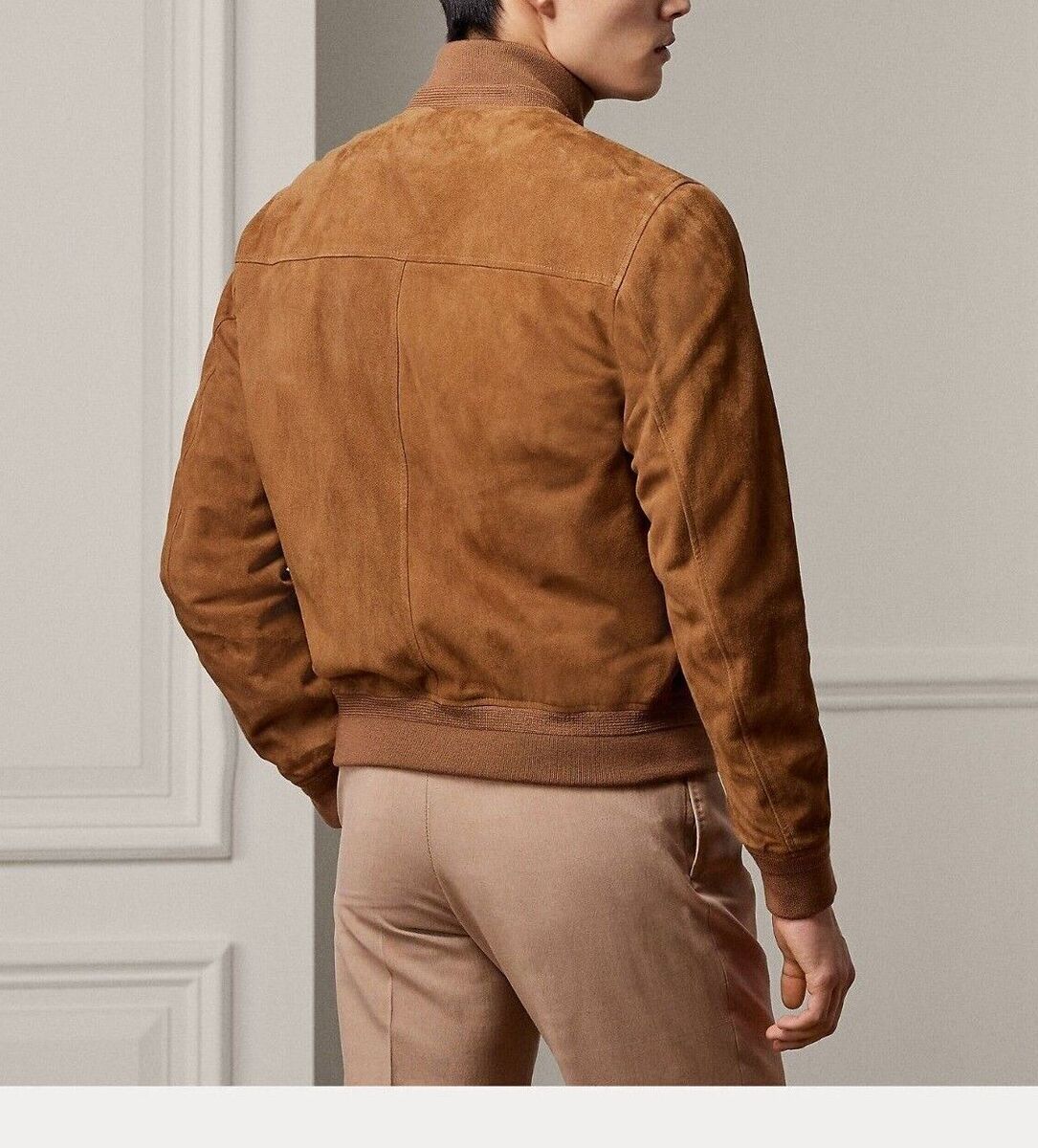The image captures a promotional photograph of a model, presumably Caucasian, wearing a stylish brown leather jacket and beige cloth pants. The model is facing away from the camera, with his head turned to his right, revealing a partial profile of his face, including his nose and mouth. His left hand is either in his pocket or obscured near his thigh while his right hand hangs down naturally. The setting features a plain white wall and a white door in the background, with no additional objects in the scene. The model's outfit, combined with the minimalistic background, draws attention to the fashionable and comfy nature of the brown leather jacket.